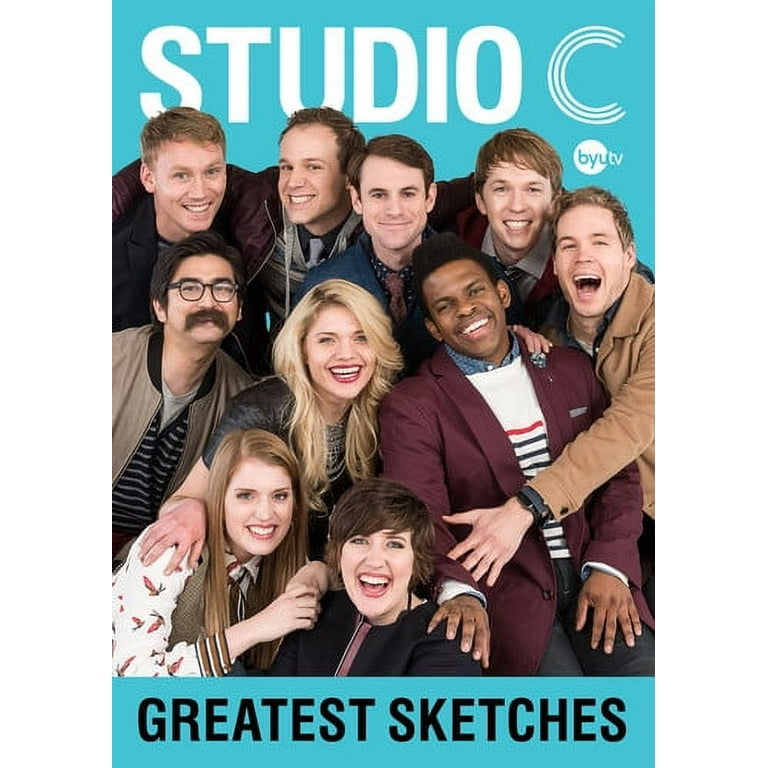The poster for the TV show "Studio C" on BYUtv features a cheerful group of actors, all closely huddled together with a mix of hugs and arms on shoulders, symbolizing their camaraderie. The backdrop is a bright teal color, and the ensemble includes ten people of mostly white ethnicity, with notable diversity in hair color, including one prominently positioned woman with very blonde hair. Arranged in three rows, the group consists of five men standing in the back row, one man sitting, and another male and female leaning in the second row, and two seated females upfront. The text "Studio C" is displayed prominently in white at the top, while "Greatest Sketches" is written in bold black letters at the bottom. Additionally, the BYUtv logo is subtly positioned beneath the "C" in "Studio C," encapsulated within a small white circle.